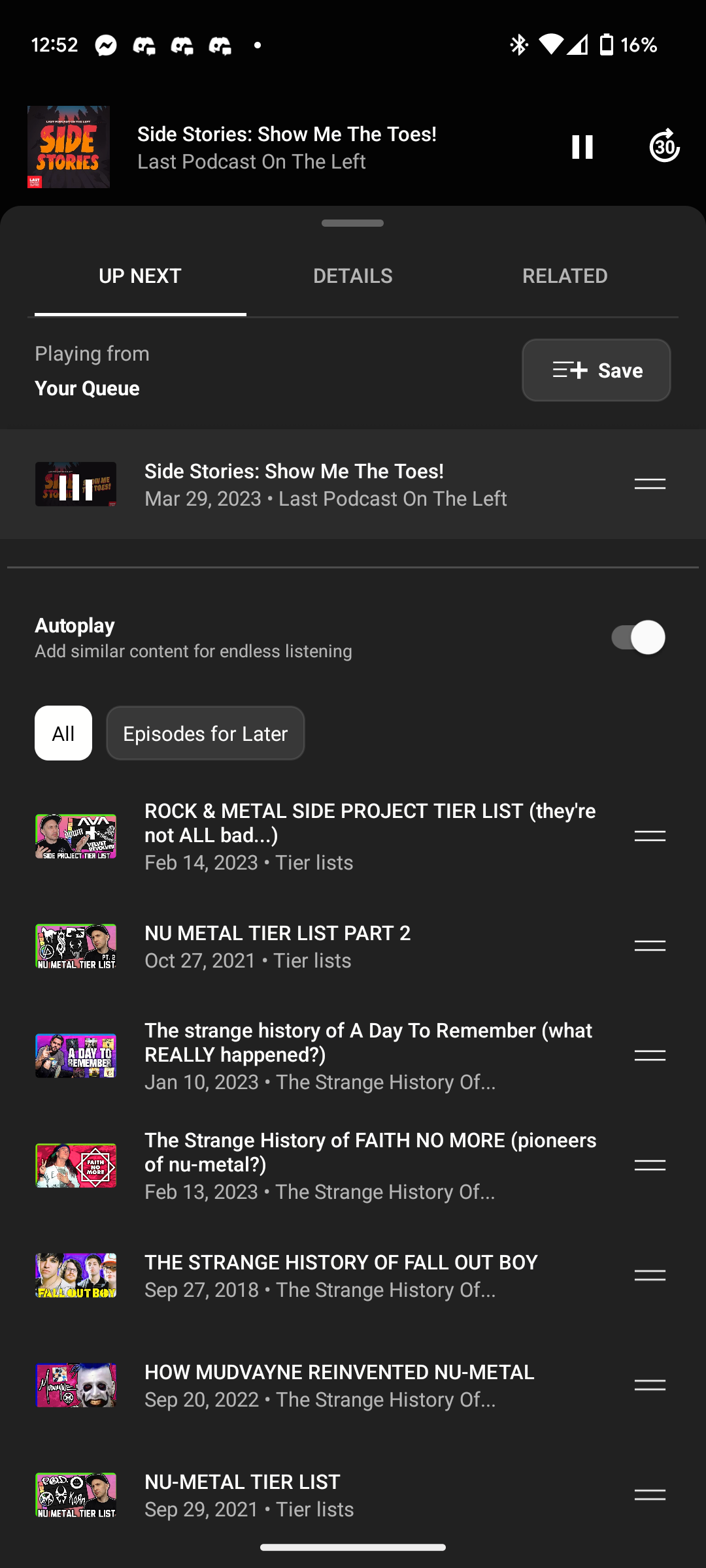The image is a screenshot taken from an unknown app or website, featuring a dark background with white text. At the top of the screen, there is a timestamp of "12:52". Below the timestamp are three Discord icons followed by another icon, which is unclear. On the right side of the top bar, there is a Bluetooth symbol, full Wi-Fi signal, strong phone signal, and a battery indicator showing only 16% remaining.

The main content of the screenshot starts with "Stories" and "Side Stories". Under these headers, there is an option labeled "Show me the toes", followed by an "Ew" reaction. In gray text, it states "Last Podcast on the Left". On the right side, there is a pause button and a 30-second skip-ahead button, both in white. Underneath, "Up Next", "Details", and "Related" options are listed.

The screenshot also displays a long list of podcasts queued for autoplay, which are difficult to turn off in Spotify, causing frustration. The queued podcasts include:
1. "Rock and Roll Side Project Tier List"
2. "Nu Metal Tier List Part Two"
3. "A Strange History of A Day to Remember: What Really Happened?"
4. "A Strange Day of Faith No More: Pioneers of Nu Metal"
5. "Strange History of Fall Out Boy"
6. "How Mudvayne Reinvented Nu Metal"
7. "Nu Metal Tier List"

The term "Nu" in "Nu Metal" appears unfamiliar to the viewer, who does not listen to metal music, adding a bit of personal frustration and confusion to the description.